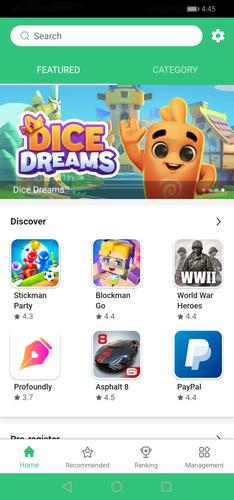The image is a detailed screenshot of a mobile app interface. At the very top, there's a black rectangular toolbar displaying a high battery level and the time, which reads 4:45. Below this, a green section features a white rounded rectangular search bar in the center, adorned with a magnifying glass icon and the word "Search." Adjacent to the search bar, there's a daisy-like flower icon. 

Underneath this green section, a prominent advertisement for the game "Dice Dreams" captures attention. The game's logo is in bold, capital letters with a blend of purple, orange, and white colors. The background showcases animated buildings, and an adorable animated character resembling a carrot with a pointed top is waving with a cheerful smile.

Proceeding further, the background transitions to white, hosting six icons and a text label "discover" with a right-pointing arrow beside it. Below this, two rows of different game recommendations are displayed. The first row includes "Stickman Party," "Black Man Go," and "World War II: World War Heroes." The second row features "Profoundly," "Asphalt 8," and "PayPal," although PayPal is not a game but has been suggested similarly.

The final section of the screenshot is a menu bar with options labeled "Home," "Recommended," "Ranking," and "Management." At the very bottom, within a green rectangle, are navigation buttons: an arrow button presumably for going back, a central button for the home screen, and another button for minimizing the interface.